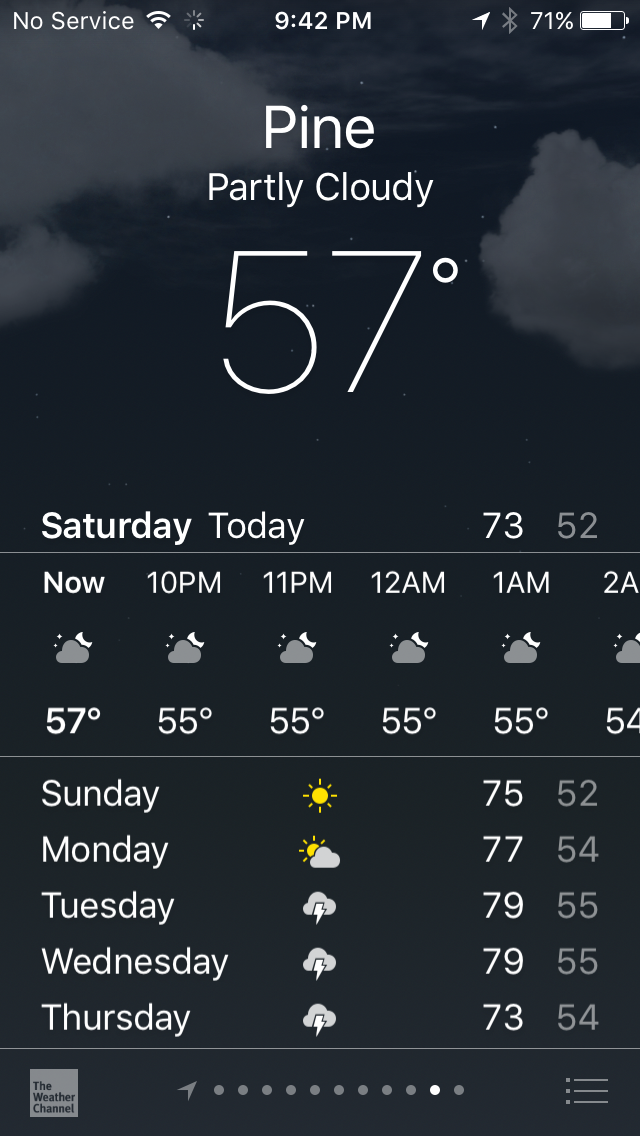This is a vertically aligned screenshot of a weather app on a cell phone. At the top, the notification bar displays "No Service," a Wi-Fi signal icon, and the time, 9:42 p.m. On the right side of the notification bar, the battery level is shown as 71%. Below the notification bar, the app's display reads "Pine" in white, indicating the location. Under the location name, it says "Partly Cloudy," followed by a large "57°" centered beneath it. 

Immediately below these details, the app shows the day's high and low temperatures, "73°/52°," labeled under "Saturday" and "Today." Below this, a timeline of hourly temperatures starts with "Now" and includes 10 p.m., 11 p.m., 12 a.m., 1 a.m., and 2 a.m., showing temperatures of 57°, 55°, 55°, 55°, 55°, and 54°, respectively.

Further down, a column lists the upcoming days: Sunday, Monday, Tuesday, Wednesday, and Thursday along with their associated weather icons and daytime/nighttime temperatures. Sunday displays a sun icon with temperatures 75°/52°, Monday shows a sun with a cloud (77°/54°), Tuesday has a thunderstorm icon (79°/55°), Wednesday shows another thunderstorm icon (79°/55°), and Thursday also shows a thunderstorm icon (73°/54°).

The background of the app features a black color with some scattered gray clouds across the middle. At the bottom left corner, the screen indicates the app source, "The Weather Channel."